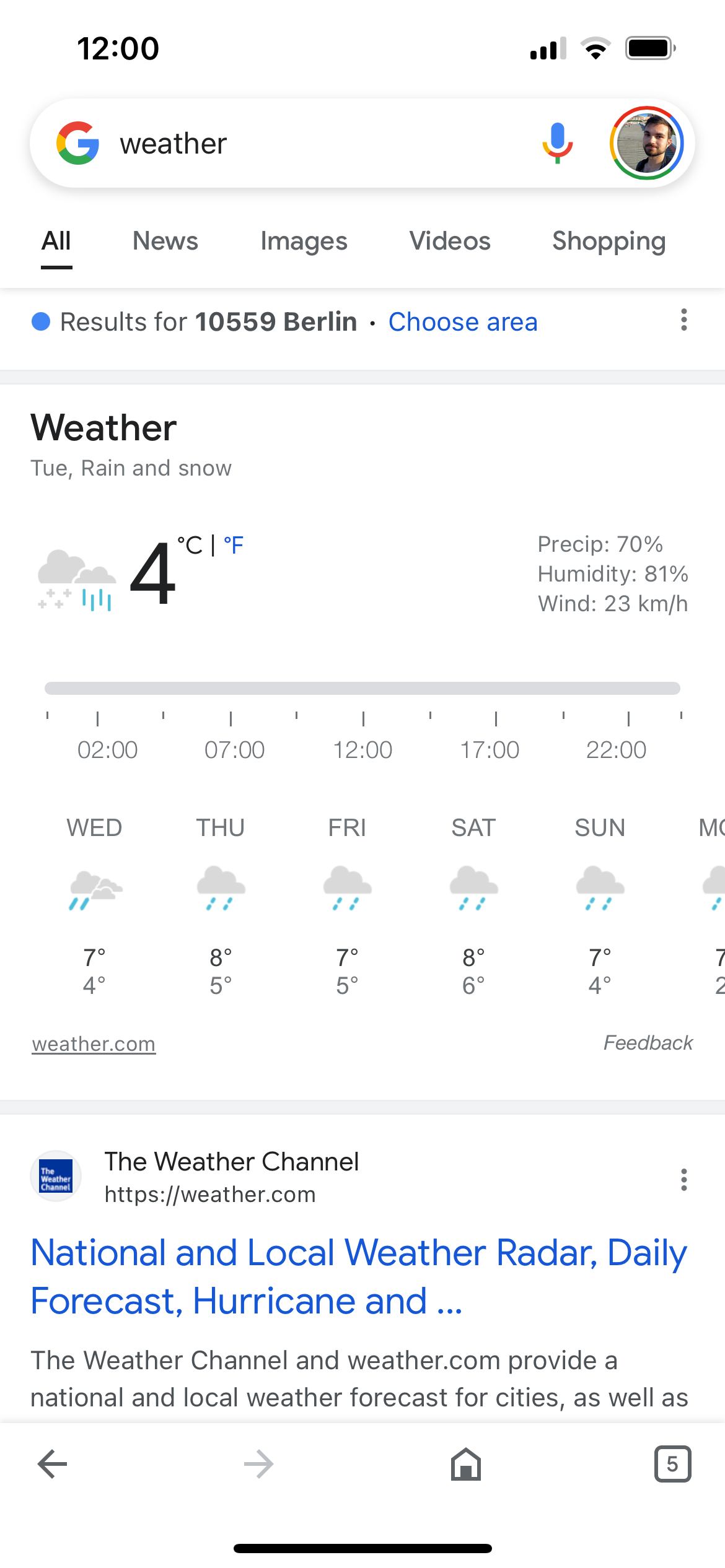The image is a screenshot displayed in a long, single column in portrait mode, set against a white background. In the top-left corner, the time reads 12:00, while the top-right corner shows a fully charged battery icon. Beneath these, there is a search bar where "weather" has been typed in Google Chrome. To the right of the search bar, there is an avatar icon representing a user's Google account.

The navigation tabs for "All," "News," "Images," "Videos," and "Shopping" follow, with "All" being underlined, indicating the active tab. Below these tabs, the search results specify the location as "10559 Berlin," with an option to choose a different area in blue. The main weather summary indicates that on Tuesday, the weather will be rainy and snowy with a temperature of 4 degrees Celsius, clearly pointing to Berlin, Germany, as the location.

A detailed weather overview on the right shows a 70% chance of precipitation, 81% humidity, and winds blowing at 23 kilometers per hour. A time chart is included, marking intervals from 2 AM to 10 PM (2, 7, 12, 17, 22), covering the entire day. An extended forecast displays the weather for Wednesday through Sunday, with Monday partially cut off, suggesting horizontal scrolling is needed to view more.

At the bottom, there is a reference row with snippets from "The Weather Channel" and "Weather.com," featuring a live link in blue text to "National and Local Weather Radar, Daily Forecast, Hurricane ..." for more detailed weather information for the upcoming week.